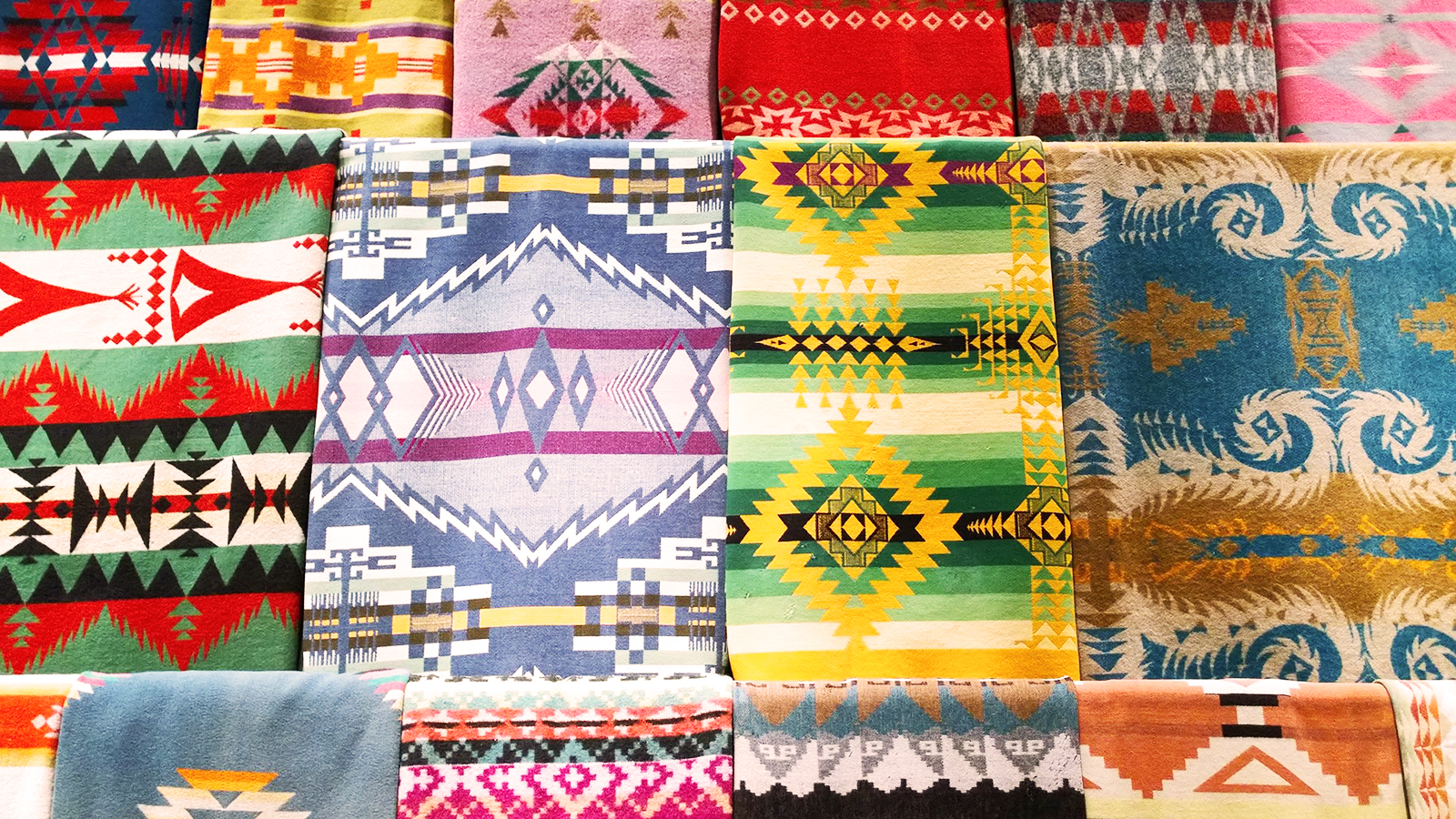The photograph showcases an array of beautiful textiles hanging side-by-side over rods, arranged in three rows. Each textile is unique, featuring a variety of vibrant colors and intricate geometric patterns reminiscent of Native American designs. On the right side, one piece stands out with its gold and blue colors, adorned with a central blue diamond framed by a white feathery swirl and arrowhead shapes. Another notable textile has alternating dark and light green horizontal stripes interspersed with white, and is overlaid with a yellow jagged-edged diamond containing an intricate design. There are textiles with colors ranging from green, red, and black, to blue, yellow, and burgundy. More textiles showcase stripes in green and intricate yellow geometric patterns, while others feature combinations of blues, creams, and golds. From grays and oranges to pinks and browns, each textile boasts a meticulously woven pattern, with many displaying diamonds, triangles, and zigzag motifs. Despite their variations, all pieces share a rich, artisanal quality, making the collection visually stunning and culturally evocative.